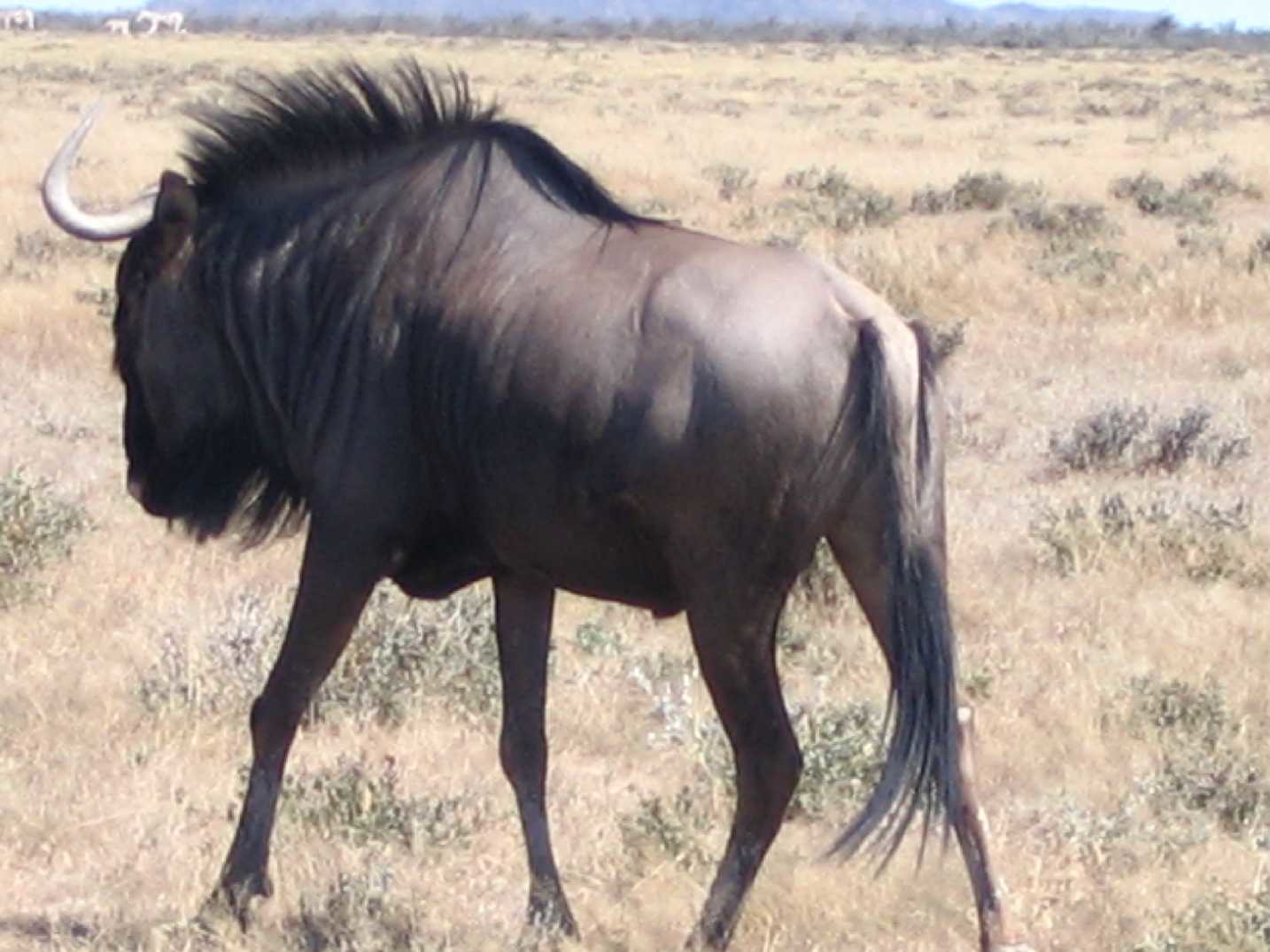This image appears to be a screenshot from a live-action video taken on an African Safari, capturing a wildebeest in a dry, grassy savannah. The wildebeest, viewed from a slight side angle with its rump near the right side of the frame and its head towards the left, exhibits typical characteristics such as a long tail and curved white horn visible on the left side of its head. It features a black mane running along its back to the hump and some fur on the underside of its mouth. The animal's body is depicted as robust rather than skinny, with a dark brown or blackish hue. The image, although somewhat blurry, shows a background filled with tan, dried-out grass interspersed with green shrubs. In the top left corner of the frame, faintly visible, are a few small white animals. The distant backdrop includes mountains with a bluish tint.